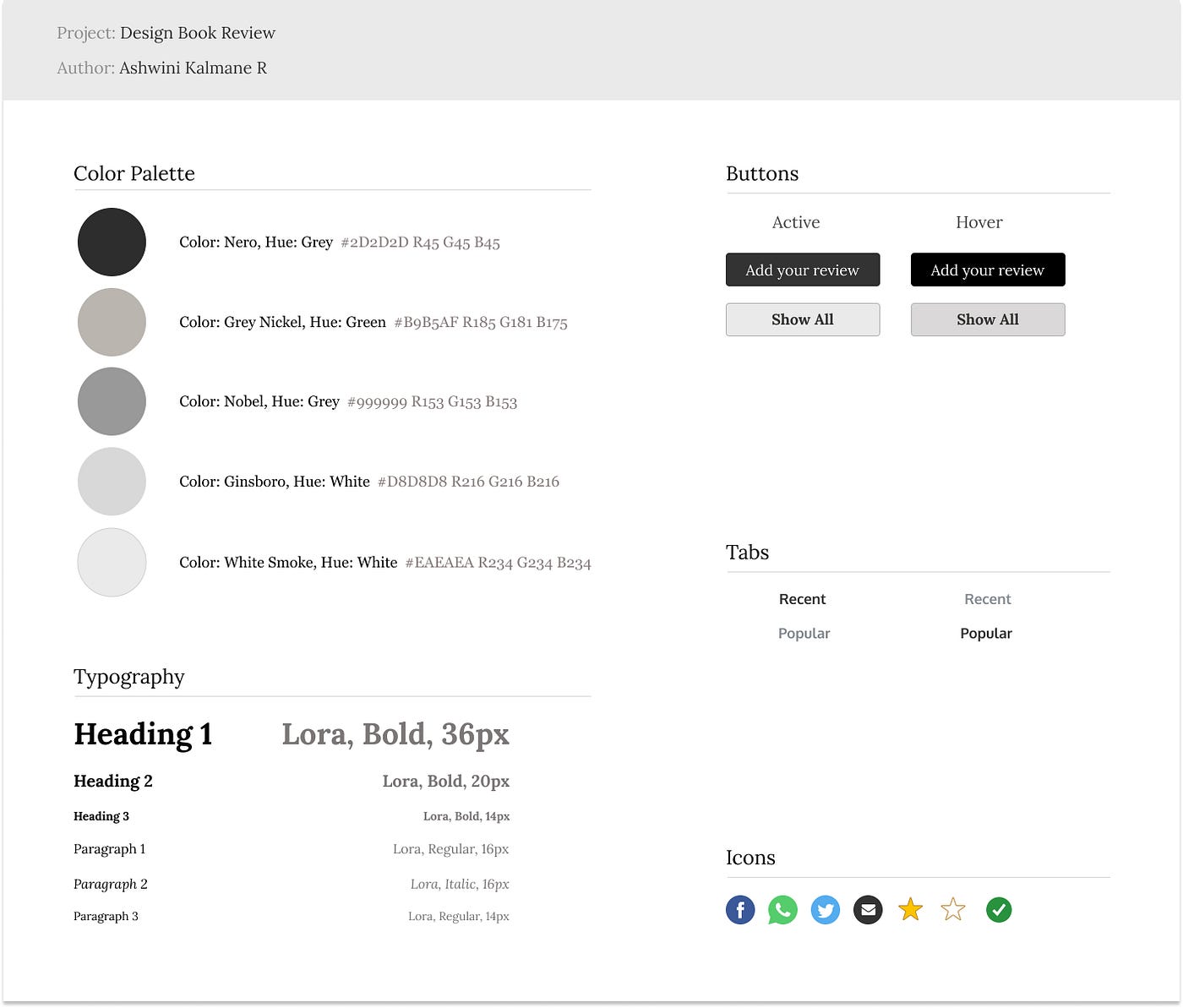This screenshot depicts a webpage specializing in book design under the project title "Design Book Review" by Ashwini Kaumaini R. The design employs a subtle, muted color palette dominated by nude tones. Among the palette, the color named Nero stands out with its greyish hue, and there are complementary hues including a greenish shade, various greys, and multiple whitish tones.

Typography is understated yet effective, using a subdued grey font. The primary heading (Heading 1) is styled in a bold Laura font at a size of 36 points. The navigation bar, recently reopened due to its growing popularity, features interactive buttons labeled 'active' and 'hover.' These buttons enable users to add a review, hover over reviews, and access all existing reviews.

In the bottom right-hand corner, there are icons for social media platforms, including Facebook and WhatsApp, among others. These icons facilitate sharing and networking for users engaged with the webpage.